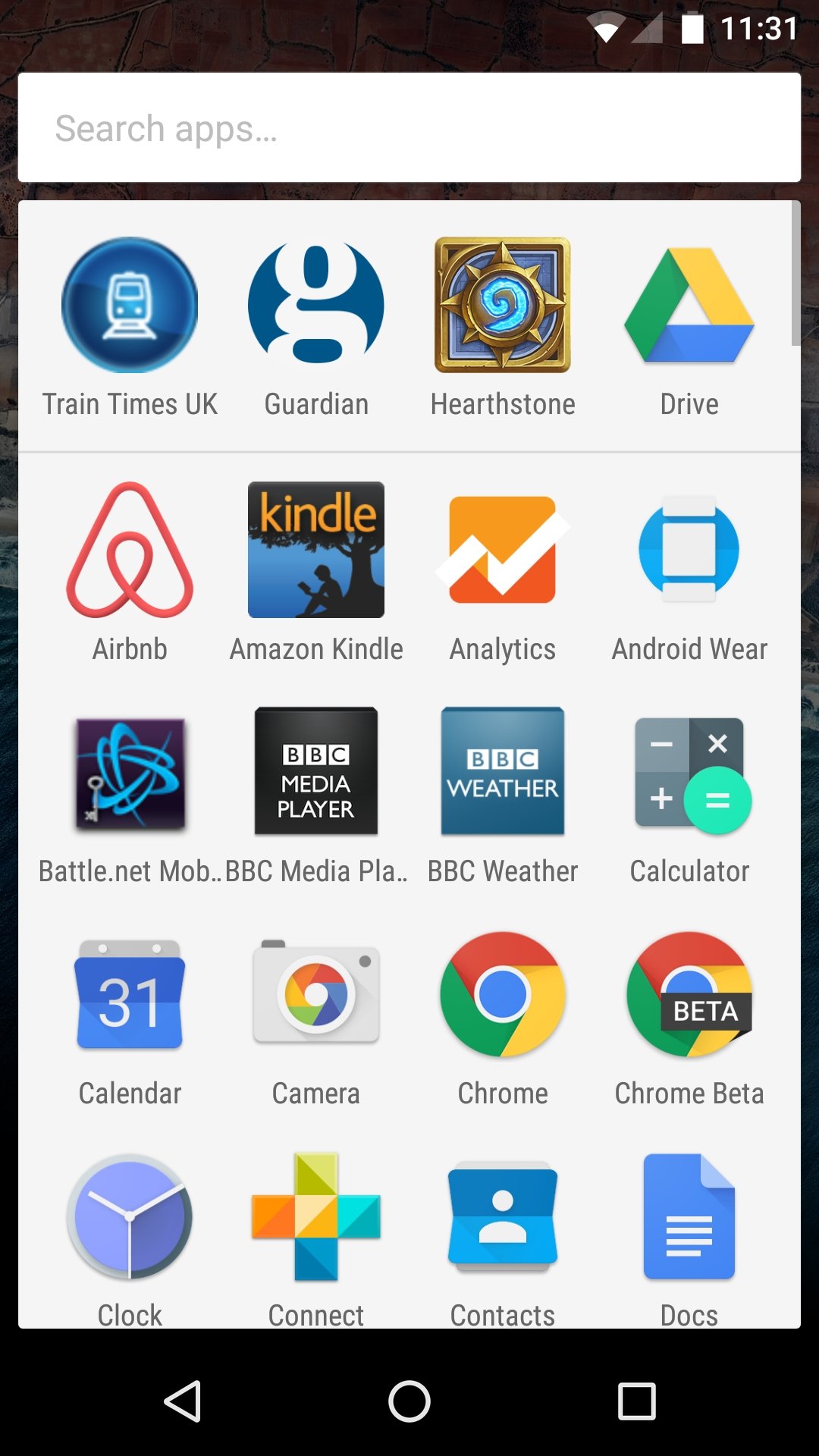This is a detailed and organized screenshot of a mobile phone interface. At the top, there's a black status bar displaying various icons for WiFi, mobile signal, battery level, and the current time reading 11:31. Directly below the status bar, there is a white search field with grey placeholder text that reads "Search apps...".

The main part of the screenshot showcases a white background filled with numerous app icons arranged in a grid format. On the top row starting from the left, the first app visible is "Train Times UK" which features a blue icon with a white train. Next is "Guardian" with its blue icon and a prominent white G. Following is the gaming app "Hearthstone", represented by a gold icon featuring a distinct blue swirl. The "Drive" app icon, similar to a recycling symbol but rendered in Google's signature rainbow colors, sits beside it.

Continuing further down, the next row begins with "Airbnb" which is symbolized by a swirl forming an A. Then there's "Amazon Kindle" characterized by an icon of a person reading beneath a tree. "Analytics" follows with its white stripe design, and beside it, the "Android Wear" app displays its icon resembling a watch band. The remaining visible apps include "Battle.net", "BBC Media Player", "BBC Weather", "Calculator", "Calendar", "Camera", "Chrome", "Chrome Beta", "Clock", "Connect", "Contacts", and "Docs", each depicted with its distinctive icon offering a visual cue of its functionality.